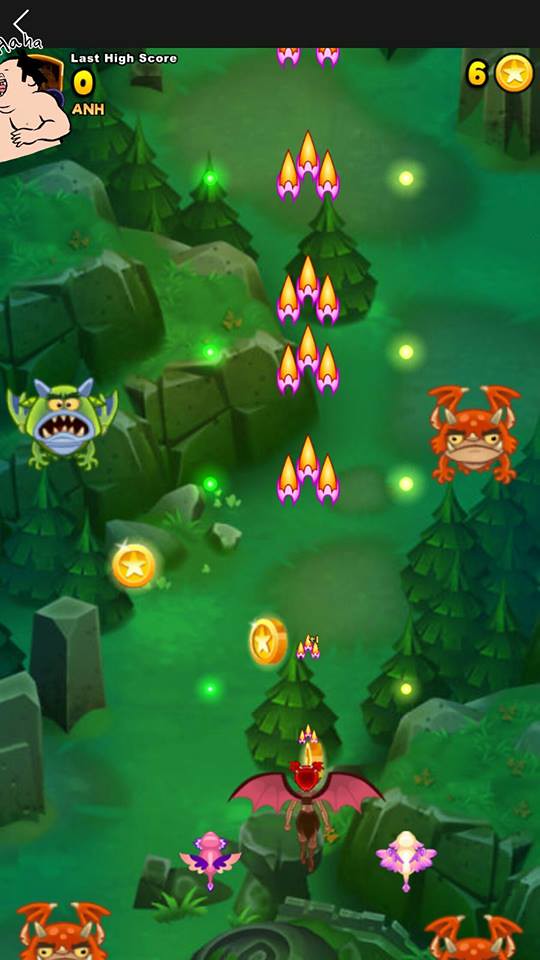The image is a detailed screen capture of what appears to be an old-school mobile video game set in a lush, green forest environment with trees, big rocks, and sparse patches of water. The forest floor is mostly covered with grass. Prominently at the center of the scene are glowing green lights, likely in-game elements or objectives.

On the left, there's a green frog-like creature standing over a mountainous area, while on the right, an orange frog-like creature mirrors this position. Below, partially visible, are two more orange frog-like figures, suggesting they might be additional characters or game assets.

Among the creatures are also a green monster with wings and an orange monster with wings, flying in the air, resembling frogs but with an almost fairy-like appearance. A distinct humanoid character with pink wings and purple hair, who might be the player’s avatar, stands facing upwards. Flanking this character are smaller, similarly pink flying figures, likely additional fairies or companions.

Scattered about the scene are several gold coins marked with stars, indicating collectible items in the game. Additionally, there are icons resembling purple aliens with fiery red heads scattered ahead of the main character. Text on the screen includes the score at the top right, which reads "6 goals," and a "last high score" noted at the top left, providing indicators of the gameplay objective and progression.